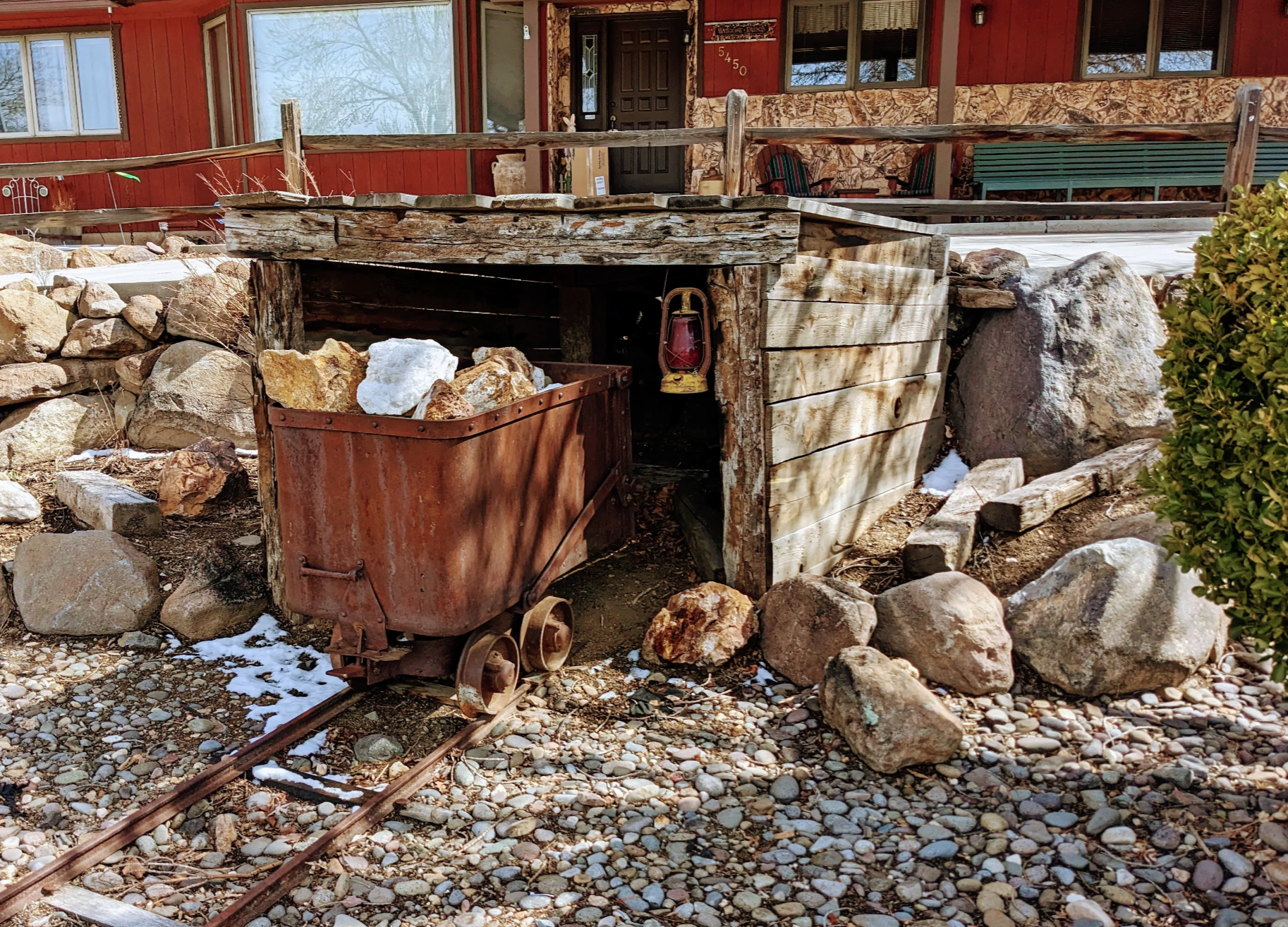The image depicts a picturesque scene featuring a cabin-like house with burnt red walls, which appear quite new, and a black door adorned with gold address numbers. In the foreground, a focal point is the mine cart positioned on rustic tracks leading into a small, wooden shed-like structure. This mine cart, with its rusty brown wheels, appears functional and is filled with large rocks of various colors, including light brown, white, dark brown, and tan stones. Surrounding the mine cart and tracks, the ground is a blend of dirt and pebbles with a hint of snow. To the left and right, beige boulders enhance the rugged ambiance.

A notable detail is the gold-trimmed, red lantern hanging on the right side of the wooden mine structure, complementing the brown slat walls of the shed. In the background, the cabin’s red building is adorned with windows reflecting surrounding trees, brown doors, and a slatted wooden fence. A green picnic bench is positioned against a brick wall, adding to the scene's rustic charm. The overall impression is that of a meticulously crafted replica of a mine shaft entrance, with attention to details such as the realistic rocks, the antiqued railway car, and the historical lantern, blending seamlessly into the picturesque landscape.